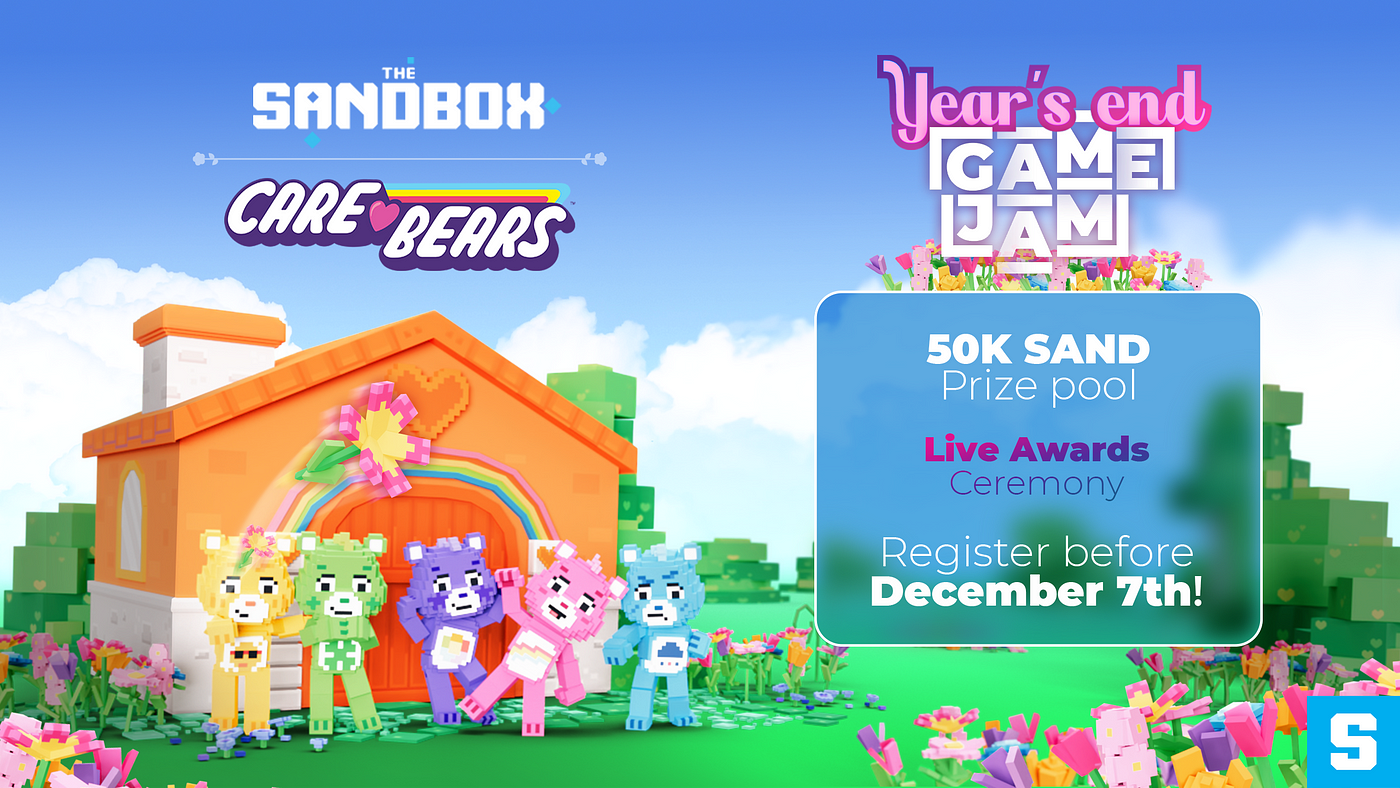This vibrant and detailed advertisement for "The Sandbox" prominently features the beloved Care Bears in a whimsical, computer-generated cartoonscape. Set against a backdrop of a blue sky with large, fluffy clouds hovering above lush green grass and dotted with trees, the scene is lively and inviting. On the top left, the title "THE SANDBOX" is displayed in all caps, with a line underneath leading to the iconic Care Bears logo. The logo is rendered in a playful, white font resembling Comic Sans, complete with a pink heart between "Care" and "Bears" and a rainbow stripe arching over the word "Bears."

In the center of the scene stands an orange brick house adorned with a rainbow arch over its door and a pink flower above it. Five charming Care Bears—colored yellow, green, purple, pink, and blue—stand cheerfully in front of the house. They represent beloved characters such as Sunshine Bear, Lucky Bear, and Stormy Bear.

On the right side of the advertisement, the event details are prominently displayed. "Year's End" is written in eye-catching pink text with a purple ombre border, while "GAME JAM" follows in bold white, all-caps letters encased in a boxy frame. Below this, the enticing "50K Sand Prize Pool" is announced, with further details in an ombre of purple and pink letters inviting viewers to a "Live Award Ceremony" and urging them to "Register before December 7th!" Completing the cheerful landscape are pixelated flowers in hues of pink, purple, and yellow scattered at the bottom, and in the bottom right corner, a small blue box featuring a white letter 'S' ties the digital theme together. This colorful and detailed ad effectively captures a sense of playful excitement, appealing to fans both young and old.